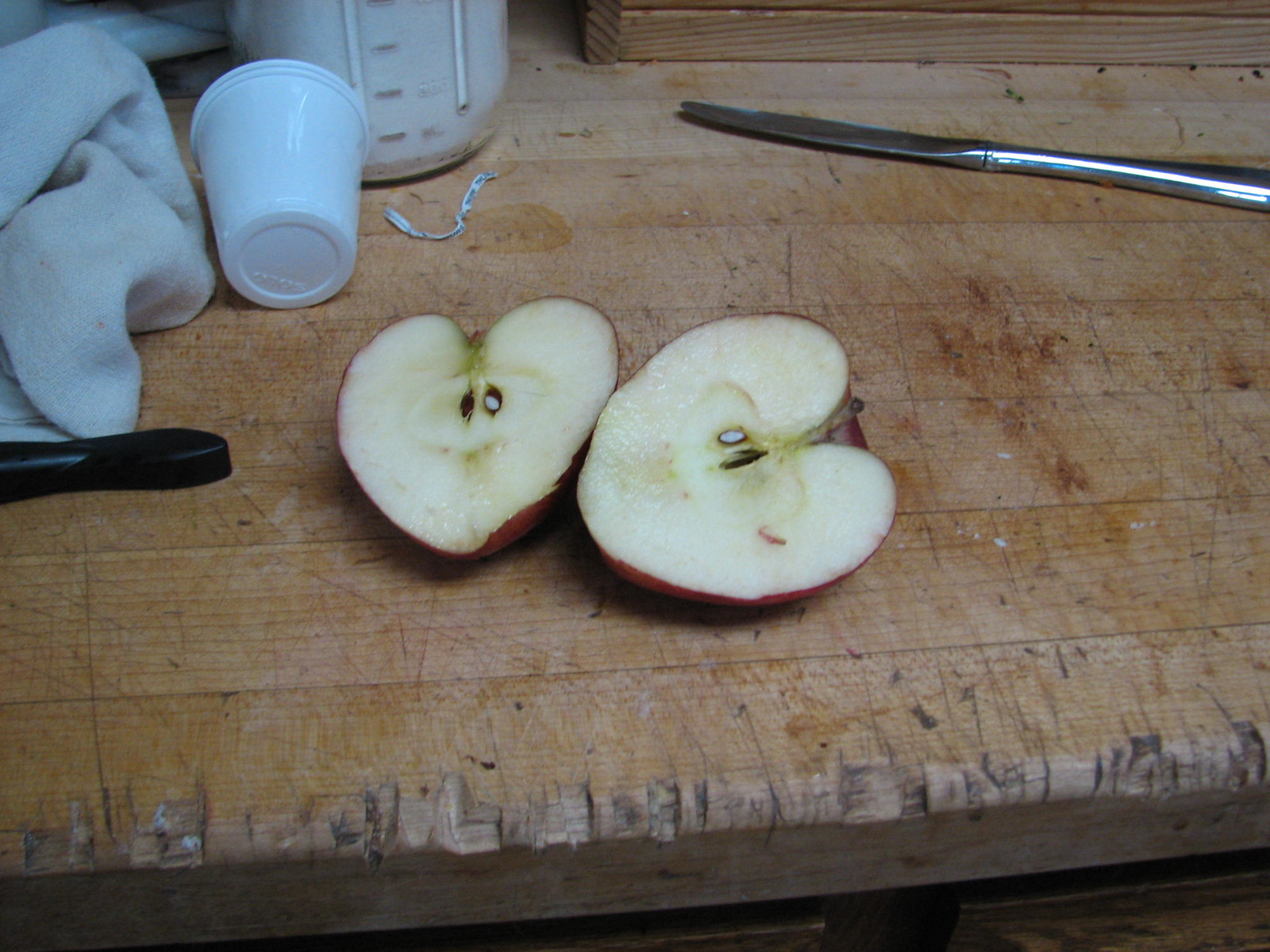This detailed photograph captures the essence of a rustic, well-used wooden countertop, which bears the marks of its history through numerous cuts, scrapes, and scratches, giving it a charming, driftwood-like appearance. The upper left corner of the countertop hosts a crumpled white dish towel, signaling frequent use. Adjacent to the towel, there are two small plastic cups, reminiscent of the disposable ones often seen at a dentist's office, neatly stacked together.

Above and slightly behind the cups, a white plastic water bottle stands upright, featuring clear measurement markings that indicate the amount of water within. This bottle adds a touch of modernity to the otherwise rustic setting. To the far right, a gleaming metal butter knife lies horizontally, ready for use.

The centerpiece of the image is an apple, precisely cut in half to reveal its fresh, moist interior. Remarkably, each half of the apple is shaped like a perfect heart, with the symmetry and vibrant white flesh drawing immediate attention. This captivating detail adds a surprising element of natural beauty to the otherwise utilitarian scene.